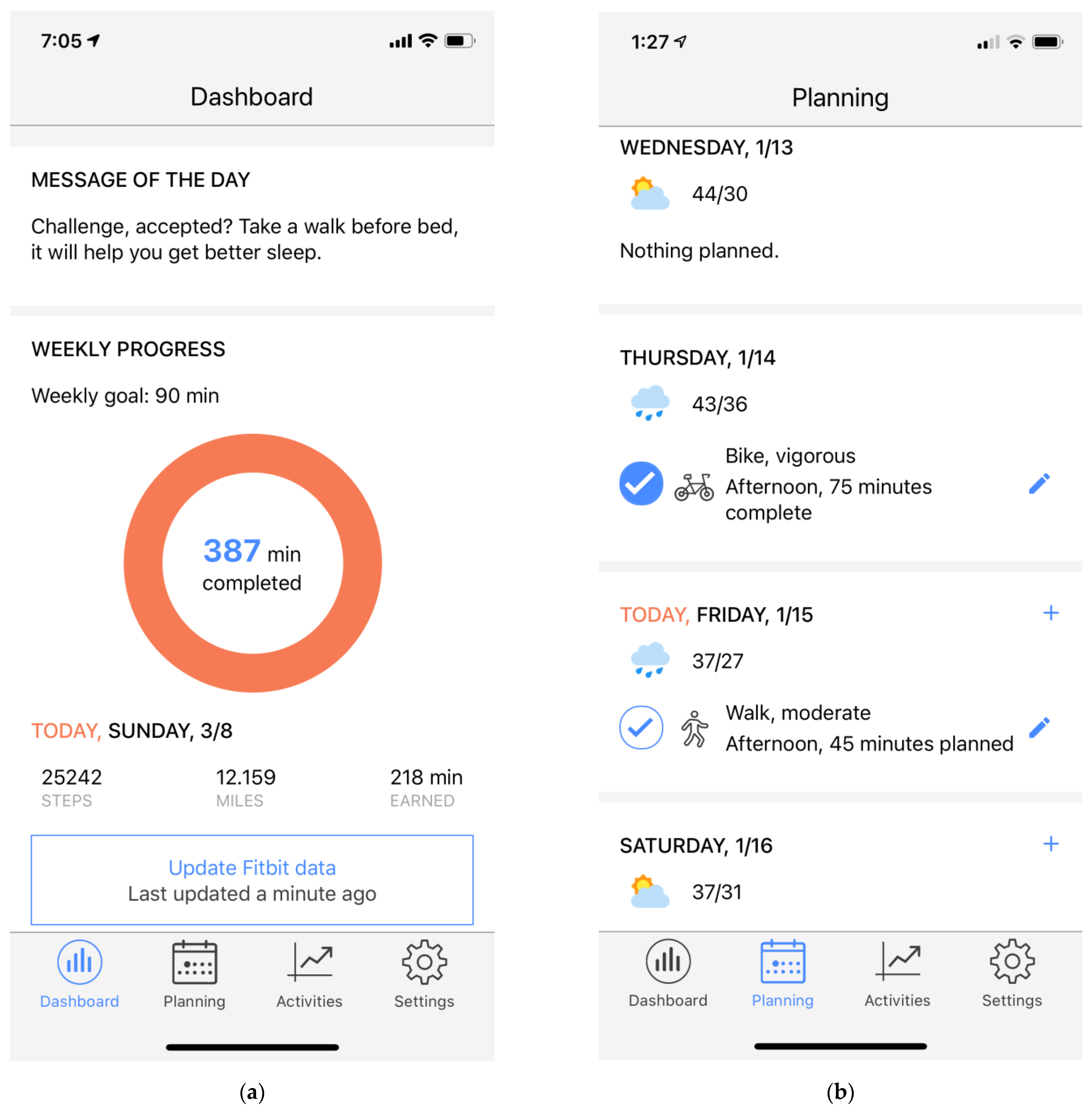The image consists of two screenshots from a planner app.

**Left Screenshot:**
- At the top, it displays the "Dashboard" section.
- Below, there is a "Message of the Day" which reads: "Challenge accepted: Take a walk before bed. It will help you get better sleep."
- Underneath the message, there is a summary of "Weekly Progress":
  - The "Weekly Goal" is to achieve 90 minutes.
  - Inside an orange circle, it shows "387 minutes completed."
- The current date is Sunday, March 8th, and the stats for the day are:
  - 25,242 steps
  - 12.159 miles
  - 218 minutes earned

**Right Screenshot:**
- The top section is labeled "Planning."
- For Wednesday (1/13), it shows:
  - 44 out of 30, with nothing planned
- For Thursday (1/14), it displays:
  - 43 out of 36, with a "Bike Vigorous Afternoon" activity, marked as completed for 75 minutes.
- For Friday (1/15), the entry states:
  - 37 out of 27, with a planned "Walk Moderate Afternoon" for 45 minutes.
- A small pencil icon is also visible, likely indicating an option to edit.

Overall, the screenshots provide a detailed view of the user's fitness and activity planning within the app.